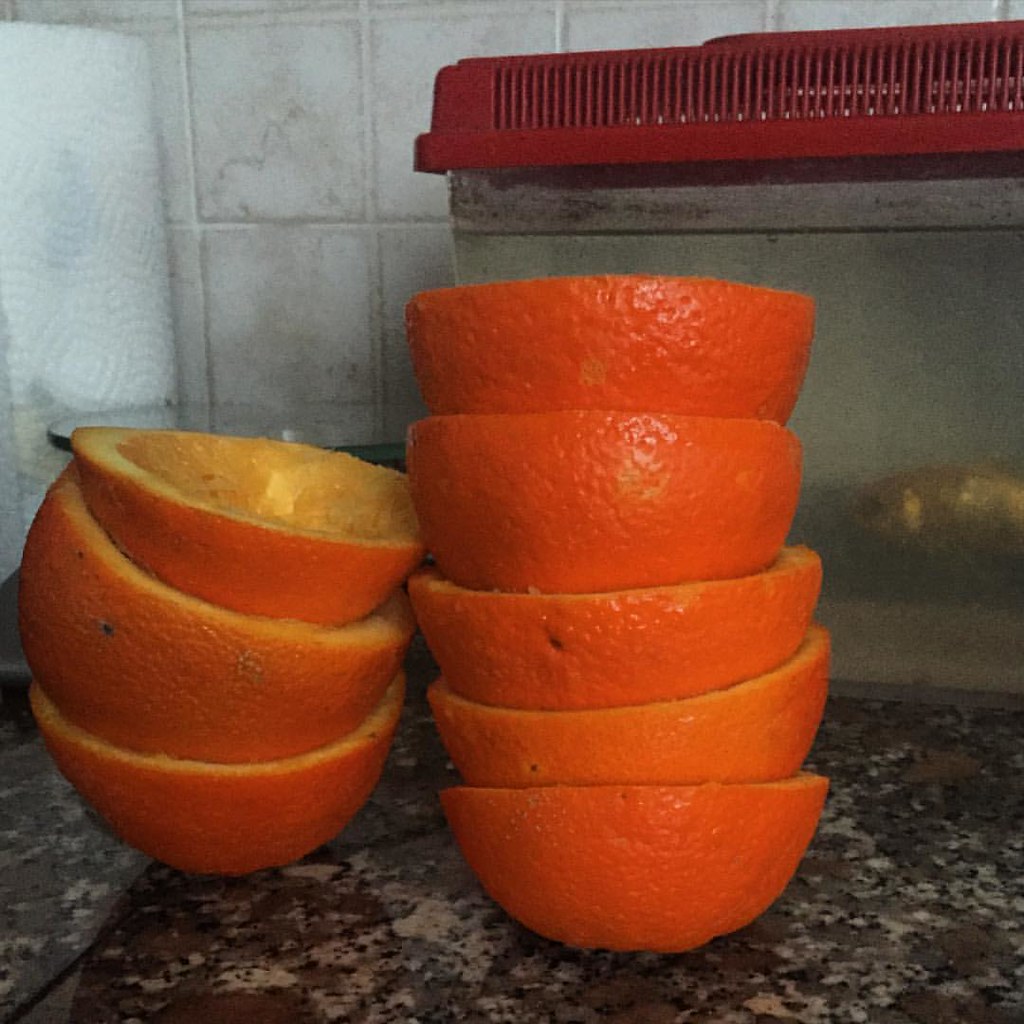The photograph is taken in a kitchen, featuring a detailed scene on a tan and black marble countertop. At the center, there are two stacks of orange halves, used for making juice. The stack on the left consists of three orange halves, and the one on the right has five orange halves, making a total of eight halves from four oranges. The thick, dimpled orange peels are stacked neatly inside one another, with the remnants of the juiced fruit visible, compressed at the top of the shorter stack. To the left in the background, there's a white roll of paper towels, and further back, a small, cloudy fish tank with a red lid and a goldfish swimming inside. The wall behind the scene is tiled with white tiles veined in gray, adding to the kitchen setting.